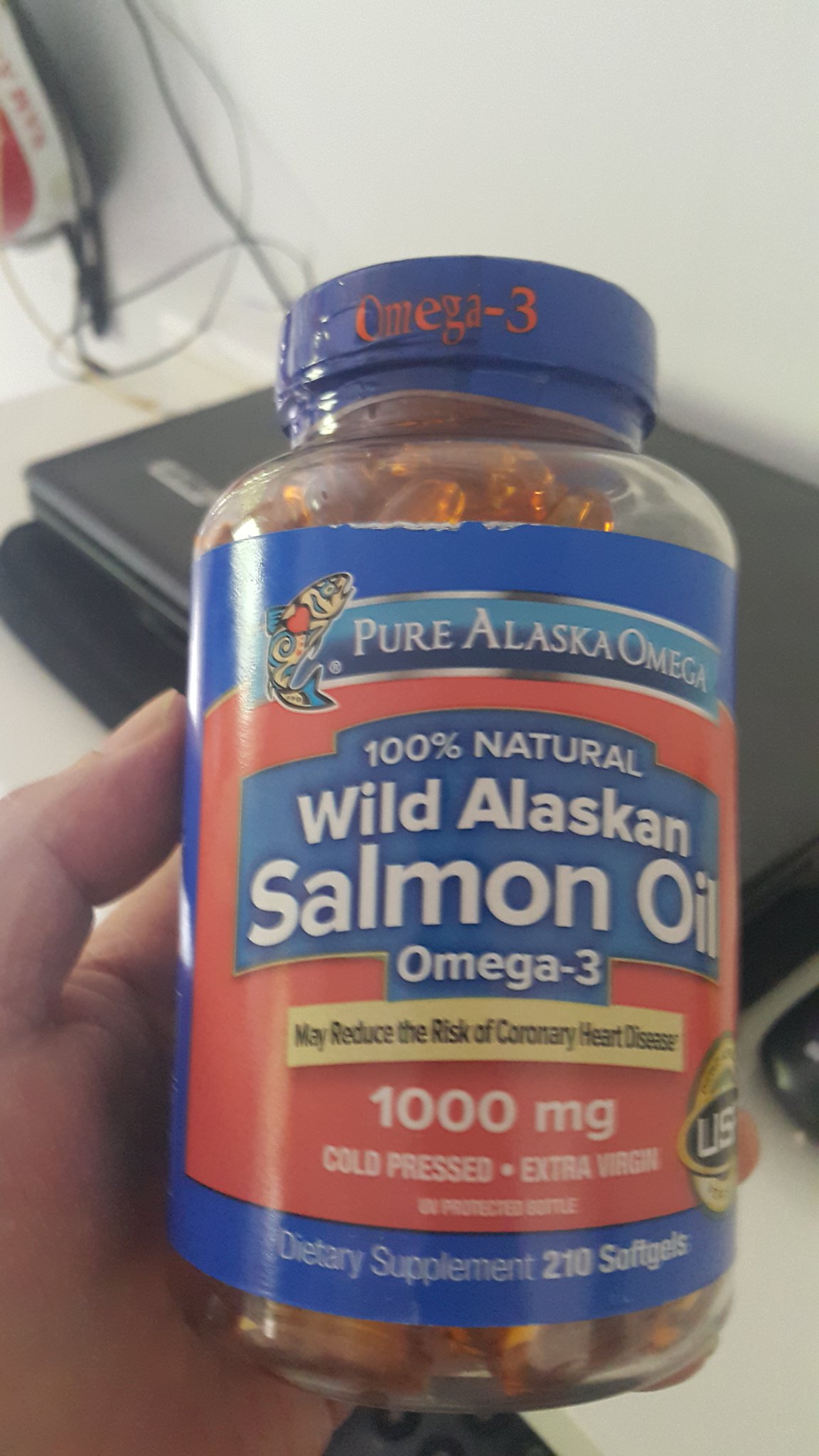The photograph features a bottle of wild Alaskan salmon oil supplements prominently displayed as the main subject. The bottle itself is made of clear plastic, topped with a blue lid. Its label, which covers most of the surface, is predominantly blue with striking pink elements. At the top of the label, a detailed drawing of a fish accompanies the text "Pure Alaska Omega" in white. Below, a large pink section holds a blue banner proclaiming "100% Natural Wild Alaskan Salmon Oil Omega 3" in bold white text. The label further details the potential health benefits, such as "May Reduce the Risk of Coronary Heart Disease," followed by the specifications "1,000 mg Cold-Pressed Extra Virgin." Finally, at the bottom, it states "Dietary Supplement 210 Soft Gels."

Through the clear container, one can see the numerous soft gels inside, filled with an orangey-pink liquid. The bottle is held in a human hand, visible from the palm up, with the thumb on the left side and the fingers mostly obscured by the bottle itself.